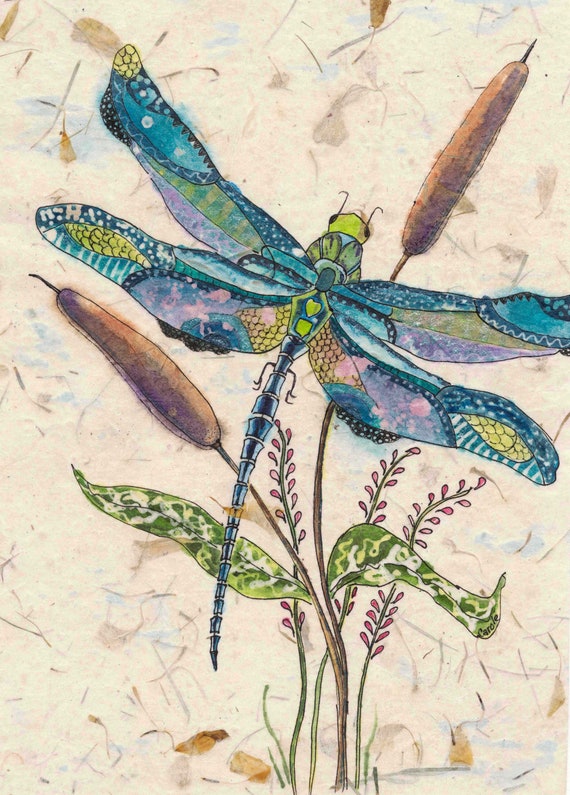This is a hand-drawn painting of a dragonfly in a rectangular frame, vividly detailed and marked by its vibrant colors and intricate design. The dragonfly, primarily a striking blue, showcases wings adorned with hues of green, purple, yellow, and hints of white. Its green head and large, dark eyes add to its distinct appearance, while its long, segmented body tapers into a tail that extends gracefully. All four of its wings are spread wide, displaying an enchanting gradient from blue to green and purple, with yellow tips.

Beneath the dragonfly, a plant emerges from the bottom of the image, featuring two green leaves and a cylindrical, brown part resembling a bulrush. Additionally, some stems with light red flowers add a touch of floral delicacy. The background is a light brown to pinkish-beige canvas embellished with various lines and random squiggles, imparting a textured and almost whimsical aesthetic. Subtle brown streaks appear in both the lower left corner and upper center, enhancing the depth and narrative of the natural scene depicted.